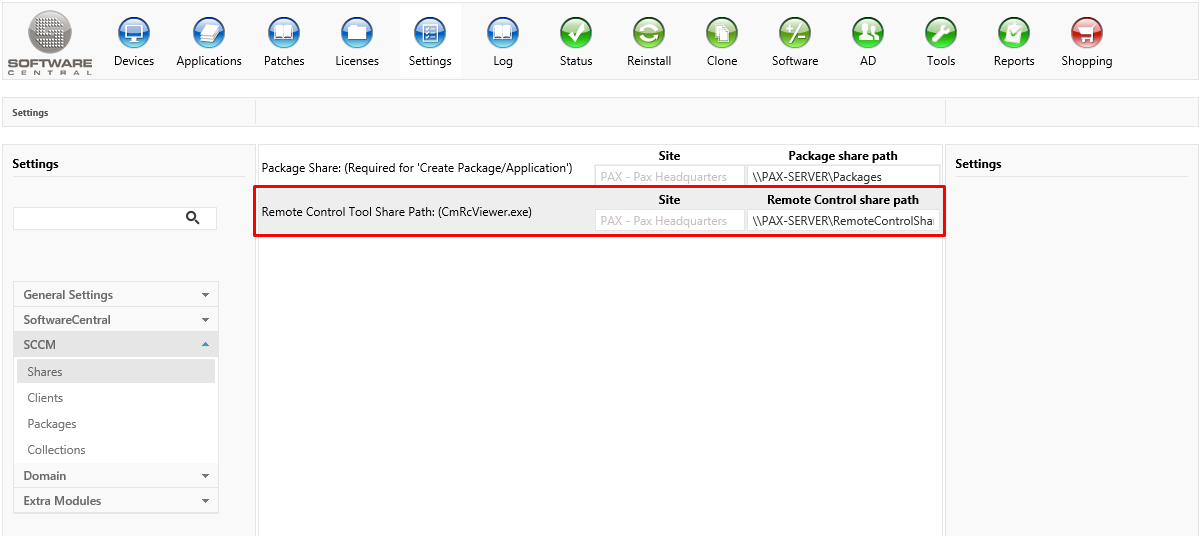The image depicts a screenshot of a detailed management interface. At the top, there is a prominent gray box with multiple tabs labeled as follows: "Software Central," "Devices," "Applications," "Patches," "Licenses," "Settings," "Log," "Status," "Reinstall," "Clone," "Software," "AD," "Tools," "Report," and "Shopping." Below this, on the left-hand side, is a navigation menu with a search box at the top. This menu lists various sections labeled: "Settings," "General Settings," "Software Central," "SCCM," "Shares," "Clients," "Packages," "Collections," "Domain," and "Extra Modules."

On the right side of the interface, there is a detailed information panel. At the top, it specifies "Package Share Required for Create Package/Application Site PAX." It continues with the label "PAX Headquarters," followed by the directory path "\\Patch-PAX-Server\Packages\Settings." Highlighted within a red rectangular box, the text indicates: "Remote Control Tool Share Path CMRCviewer.exe Site PAX," and "PAX Headquarters," with the directory path "\\PAX-Server\Remote Control\SHA." This portion of the interface ensures configuration for remote management tools and package distribution within the IT infrastructure of "PAX Headquarters."